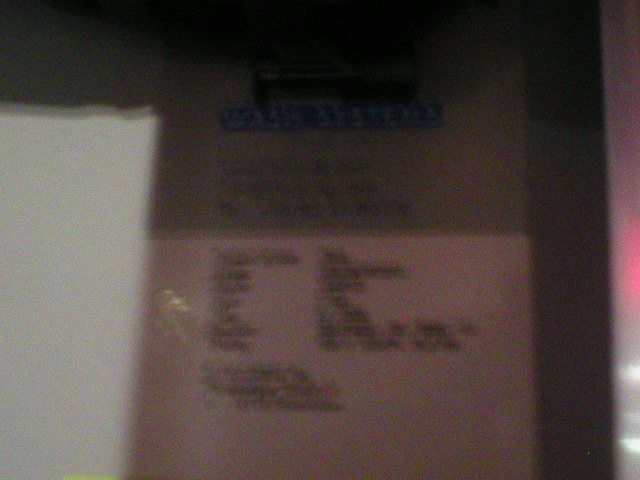This incredibly blurry, out-of-focus image appears to capture a vertical, white rectangular piece of paper, likely a receipt, set against varied surroundings. The paper is topped by a gray logo, possibly resembling a car, with an all-caps blue text directly beneath it. However, the dark shadows and poor resolution obscure the content of this text. Below this section, there's an arrangement of black text divided into a small paragraph, followed by two columns of approximately seven lines each, and another small paragraph of three lines at the bottom.

On the left side of the image, the photograph features a lighter, white rectangular shape, which might suggest a piece of styrofoam with a jagged edge, possibly seen through a glass door with wooden trim. The right side reveals a strip of silver metal adorned with reflective patches, including two white ones at the bottom and a red one halfway up. Additionally, there's a hint of a plum-colored object, potentially a window, with light shining through. Despite these various elements, the low resolution and blurriness make it impossible to discern specific details or text.